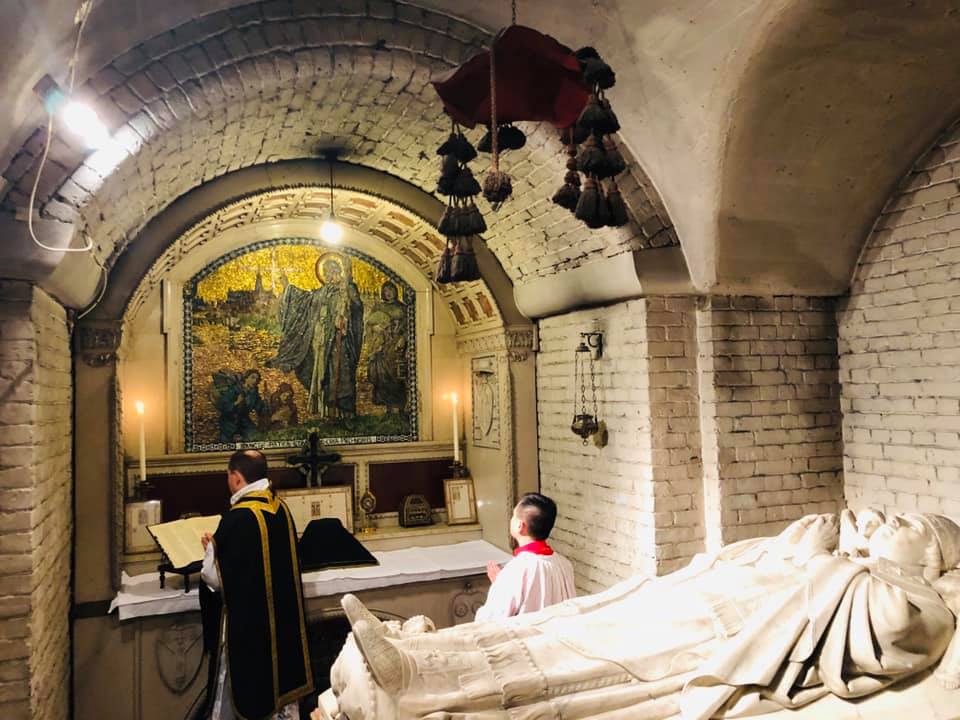The image depicts a detailed interior of a room within a religious building, likely an old-style Catholic church or monastery. The setting appears to be a side area rather than the main sanctuary. Dominating the back wall is an intricate religious picture made of tiles, rich in gold, green, white, red, and black colors. The image features a scene with a table draped in a white cloth, possibly representing an altar, with two figures—one is a man in a brown robe with a noticeable bald spot, assumed to be a priest, engaged in reading from a book, while the other figure, perhaps a deacon or altar boy, is seen bowing or praying.

The walls and ceiling are constructed of beige bricks, giving an impression of an underground or semi-enclosed space. An archway made of the same material frames the scene. A decorative object, reddish in hue and entwined with rope-like elements and possibly resembling grass, hangs from the ceiling. Near the upper left corner, two white lights add to the ambient illumination. In the lower right of the image, there is an object resembling a sarcophagus, potentially carved to look like a recumbent figure with hands in a prayer gesture. The overall palette includes shades of blue, light blue, brown, green, yellow, and red, creating a visually rich and historical atmosphere.